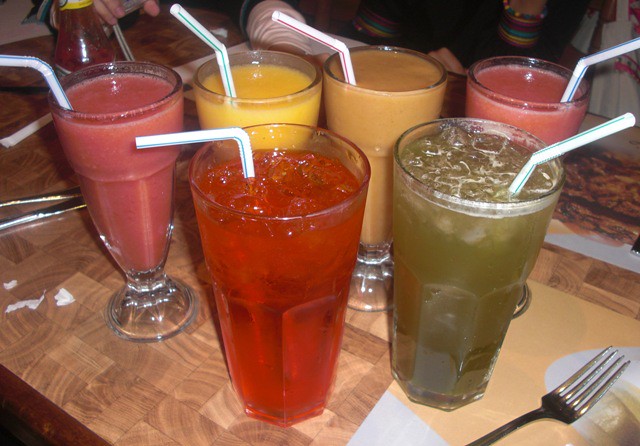A vibrant and detailed close-up photograph showcases an artistic arrangement of six colorful drinks in clear, cylindrical glasses, each with a white straw featuring colored stripes, arranged on a rustic wooden table with a textured pattern of light and dark browns. The drinks form a circular formation, with the two front glasses filled with orange and green beverages, both containing ice. Behind these, a variety of smoothies are depicted: a pink smoothie on the far left, followed by yellow, orange, and another pinkish-orange smoothie. A silver fork rests on a tan-colored placemat at the bottom right of the image. In the background, the hands and wristbands of dining individuals are partially visible, adding a casual, lively atmosphere to the scene. Additionally, a condiment bottle, possibly ketchup, appears on the far left of the table.